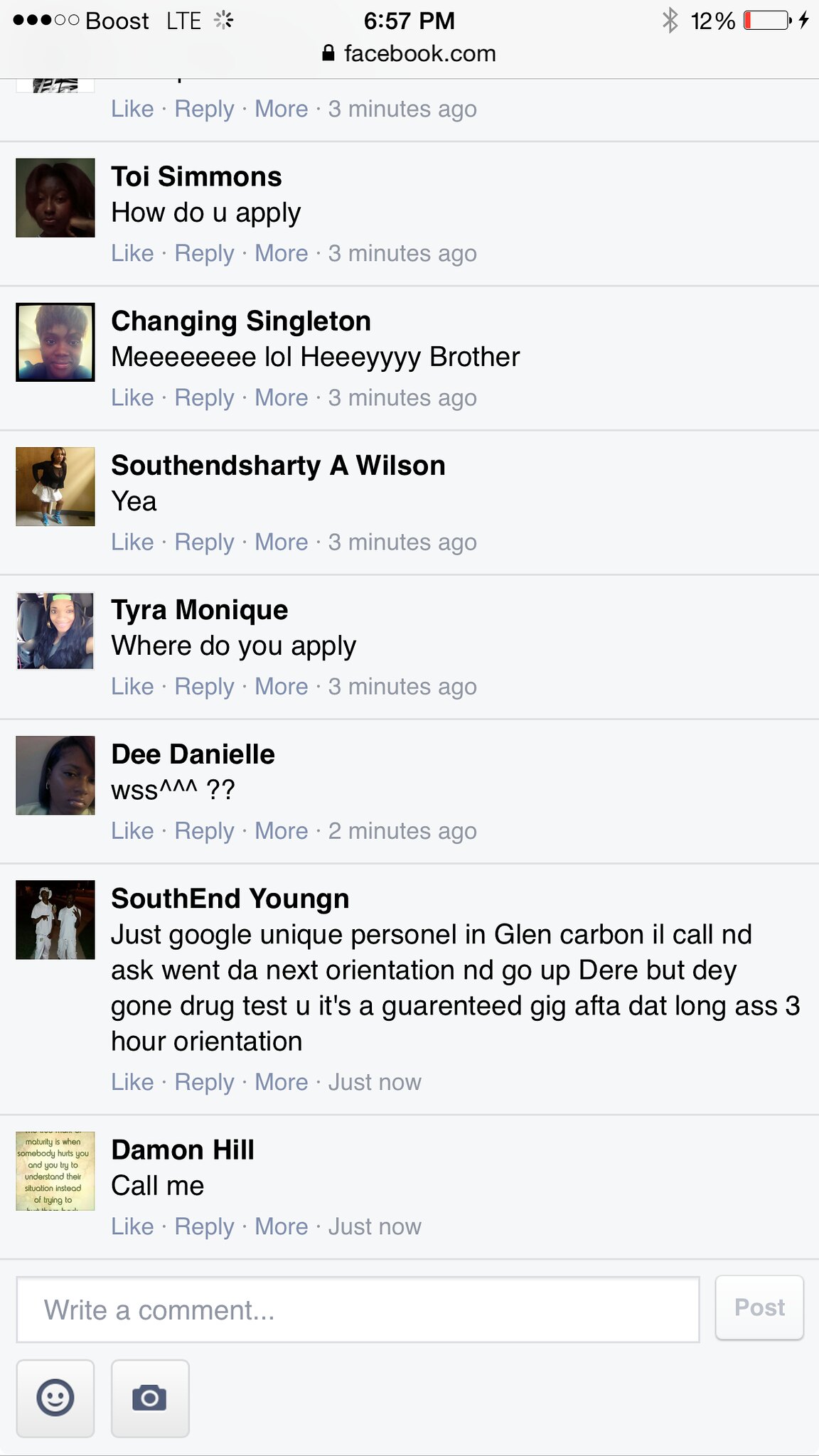The image is a screenshot of a Facebook conversation captured on a mobile phone at 6:57 PM, with 12% battery while charging. The screenshot begins with Toy Simmons asking, "How do you apply?" Chaining Singleton humorously responds, "Me, lol, hey." South End Shardy A. Wilson simply agrees with "Yeah." Tyra Monique also inquires, "Where do you apply?" D Daniels cryptically replies, "WSS, ???" South End Young N. then provides a detailed response: "Just Google Unique Personnel in Glen Carbon, IL. Call and ask when the next orientation is. Go up there, but they're going to drug test you. It's a guaranteed gig after that long 3-hour orientation." Finally, Damon Hill closes with, "Call me." The phone's background shows Boost LTE at the top.